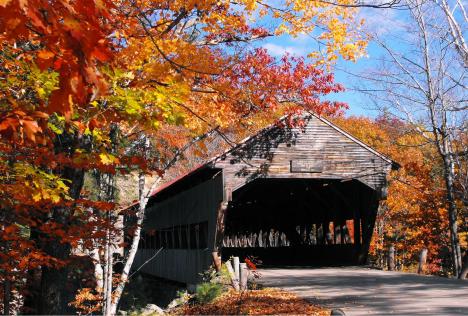The photograph captures an old, covered wooden bridge that spans a chasm, likely a river. The bridge's lower section is reinforced with asphalt, evident in the light gray portion visible in the lower right corner, allowing for vehicular passage. The structure features a triangular, dark gray wooden roof and has multiple slit-like windows, devoid of glass, that provide a glimpse inside the otherwise shadowy interior. Surrounded by a dense array of thin-trunked trees in vibrant autumn colors—orange, yellow, and brown—the scene is bathed in the light of a brilliant, sunny day, under a light blue sky dotted with clouds. The bridge appears weathered, with worn wooden panels, and though there is a sign at its entrance, its text is indecipherable. The setting underscores a serene, secluded woodland atmosphere, tinged with the characteristic hues of fall.